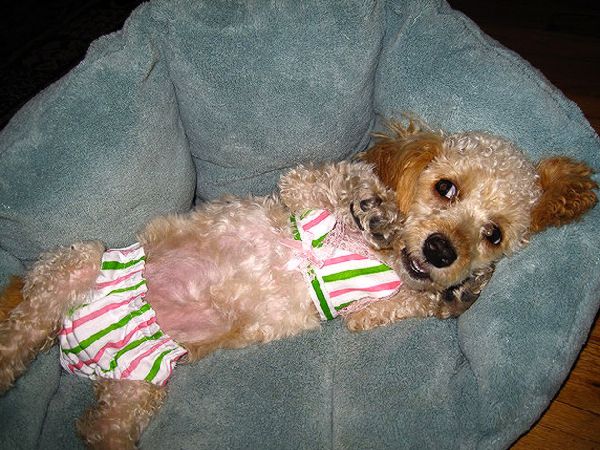In the photograph, a small dog, likely a Shih Tzu, is prominently positioned in the center, reclining on a fuzzy, swishy blue pillow. The dog is dressed in a colorful bikini, with green and pink stripes against a white background, covering both its top and bottom. The dog, featuring a coat of brown, white, and black fur, lies on its back, appearing relaxed and as if about to doze off. The setting is indoors, possibly in a living room or another area where the dog sleeps. The pillow covers most of the image, revealing just a bit of brown wooden floor in the bottom right corner. The entire photograph emphasizes the cozy and playful atmosphere, capturing the pet in a moment of rest. The image does not contain any text, and the colors visible include black, light blue, pink, green, white, beige, brown, and gray.